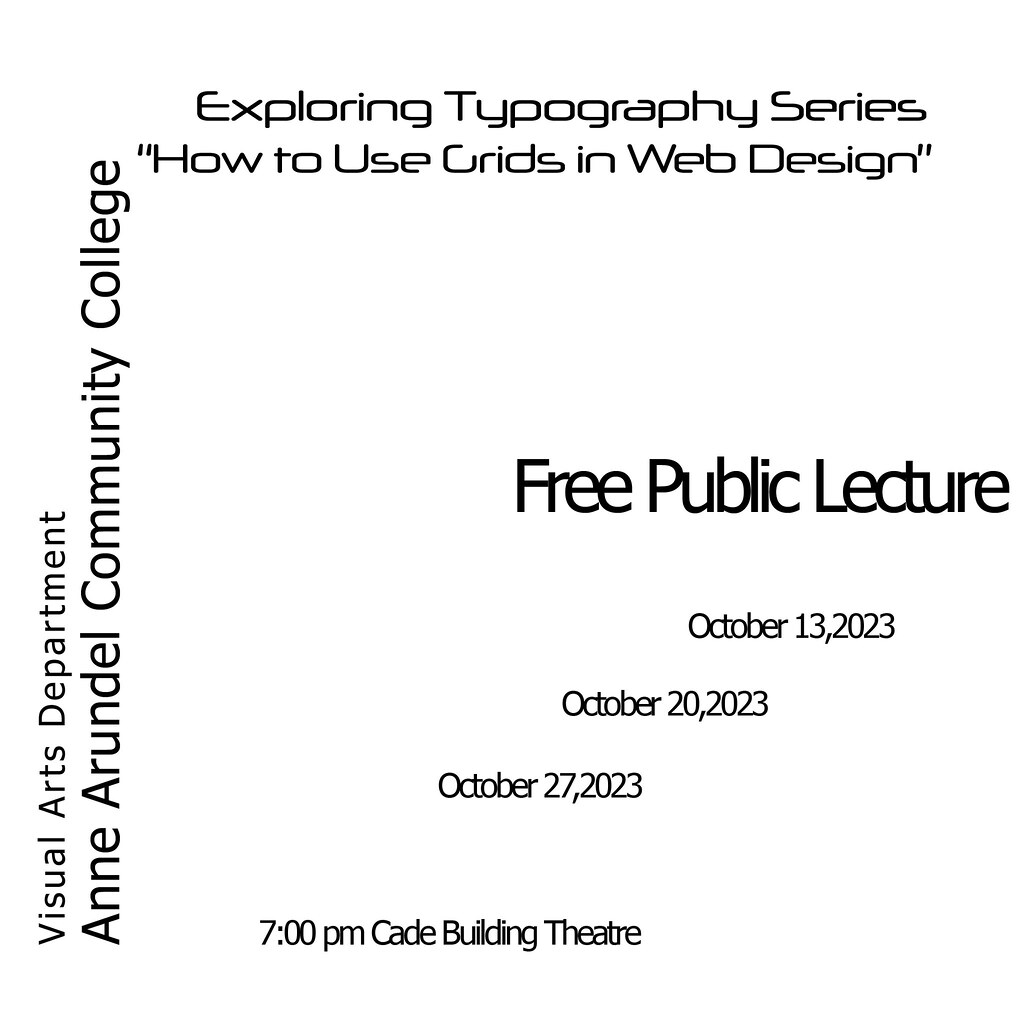The image depicts an advertisement, possibly a business card, on a white background with black ink. At the top, it reads "Exploring Typography Series: How to Use Grids in Web Design." Vertically on the left side, the text "Visual Arts Department, Ann Arundel Community College" is arranged so you need to turn your head to read it. In the middle towards the right, it announces a "Free Public Lecture" with the dates "October 13, 2023, October 20, 2023, October 27, 2023," displayed in a staggered, ladder-like format. At the bottom right, it specifies the event time and location: "7 p.m., Cade Building Theater." The simple design features no images, solely black text on a white background.